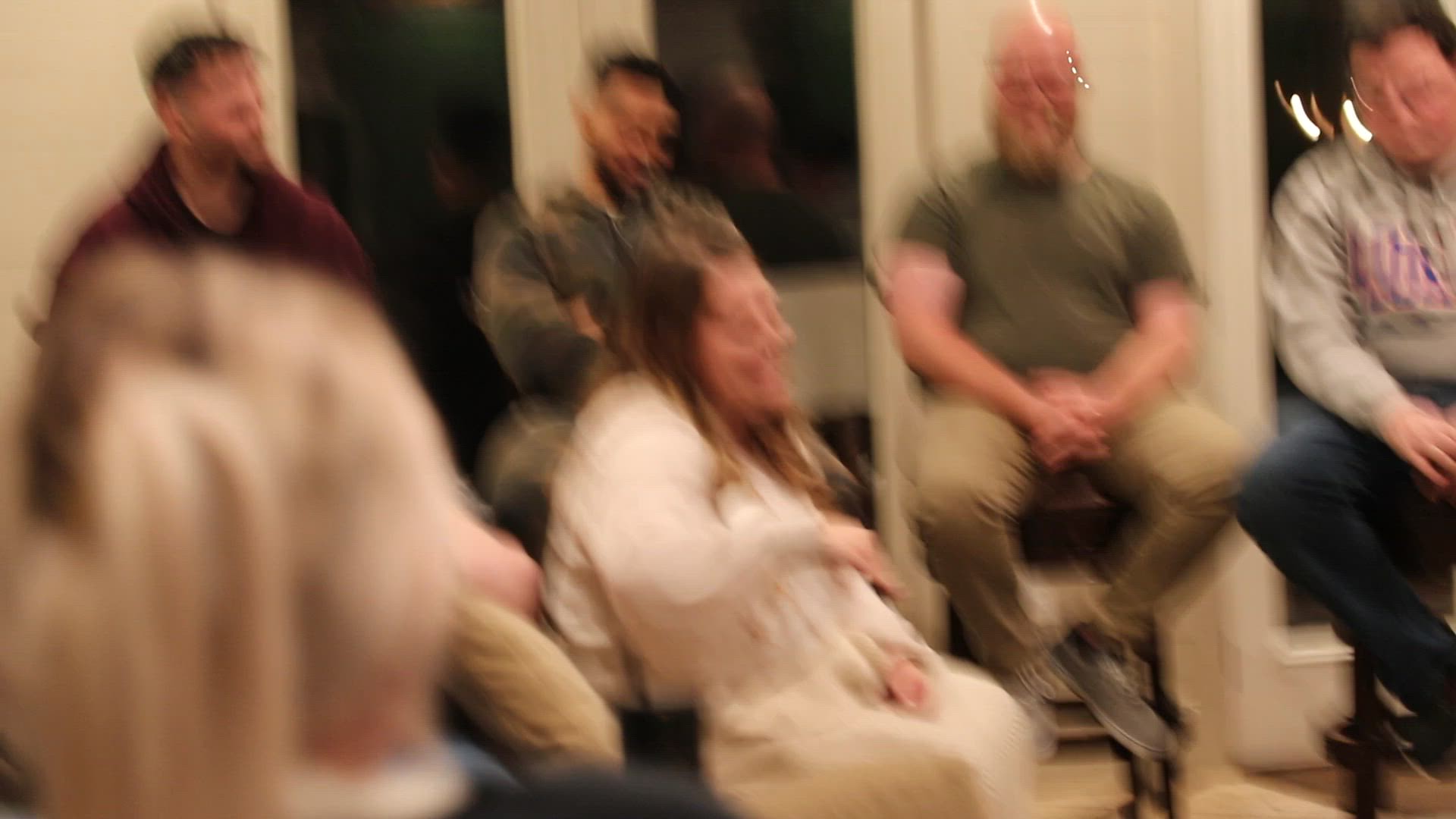The photograph depicts a group of six or seven people seated inside a room with visible windows and walls in the background. The image is notably out of focus and blurry. In the background, four men are seated in chairs; three of them have dark hair while one is bald. Two of the men are dressed in long sleeves, one in a short-sleeved T-shirt, and the attire of the remaining man is unclear. They appear to be smiling. In the foreground, a woman in a white dress is captured mid-gesture, her arm raised at an angle as she speaks animatedly, also smiling. In the very forefront of the picture, the back of a woman’s head is visible, her blonde hair styled in a puff.